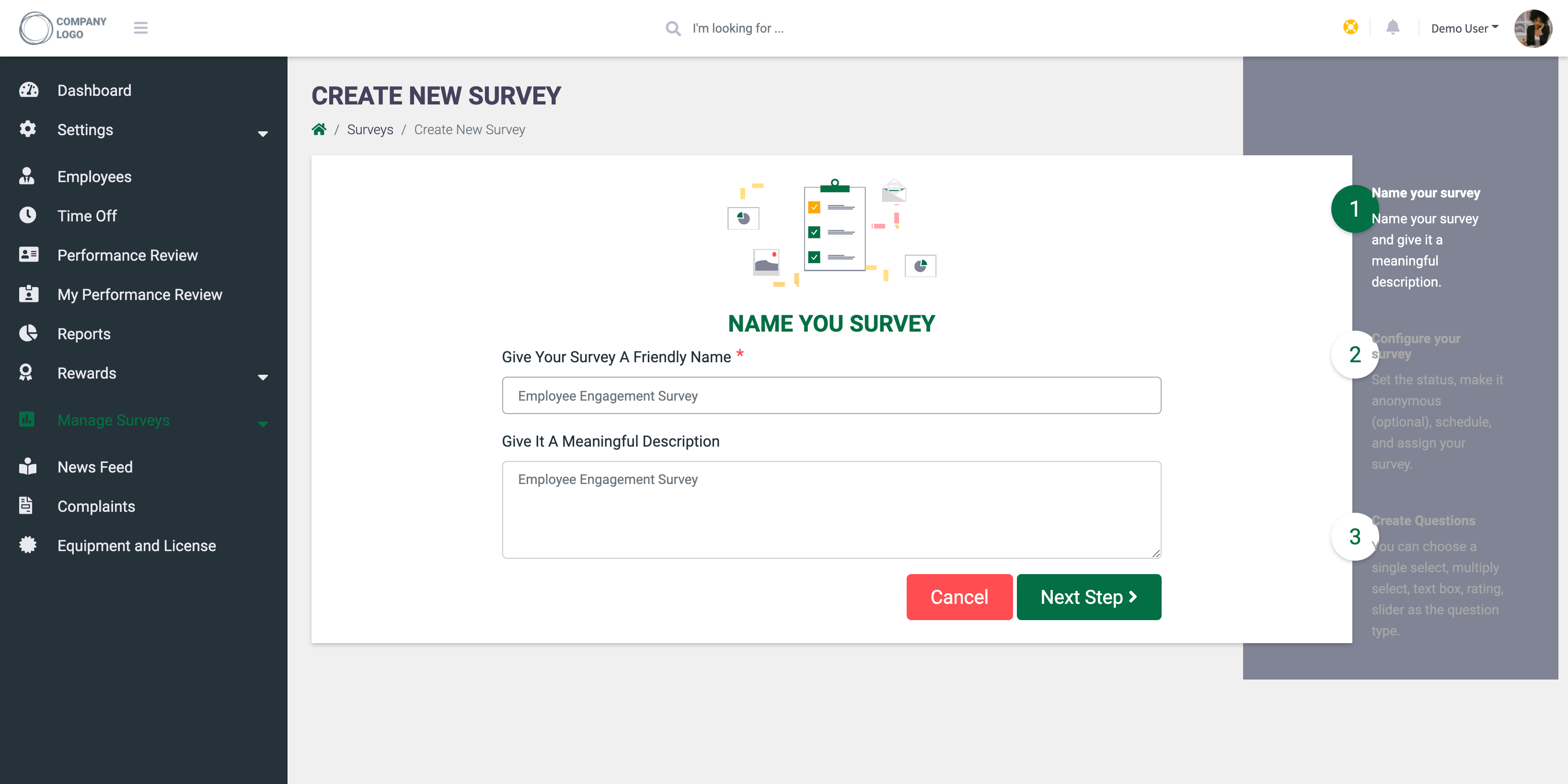This image showcases a website interface, prominently featuring the company logo in the top left corner. On the left side, a pinned navigation menu provides access to various sections, including the Dashboard, Settings, Employees, Time of Performance Review, My Performance Review, Reports, Rewards, Manage Surveys, Newsfeed, Complaints, Equipment and License, and Surveys. Specifically, the focus is on creating a new survey.

The section for creating a new survey is highlighted. There's a field titled "Name Your Survey" where users are prompted to enter a survey title—an example provided is "Employee Engagement Survey." Below, there's a space to "Give Your Survey a Friendly Name" and a description field encouraging users to "Give it a Meaningful Description." The provided description text repeats "Employee Engagement Survey."

At the bottom of this interface section, there are two buttons: "Cancel" and "Next Step." To the right, there is a clear indicator labeled "Step 1: Name Your Survey," emphasizing the importance of this initial step in the survey creation process.